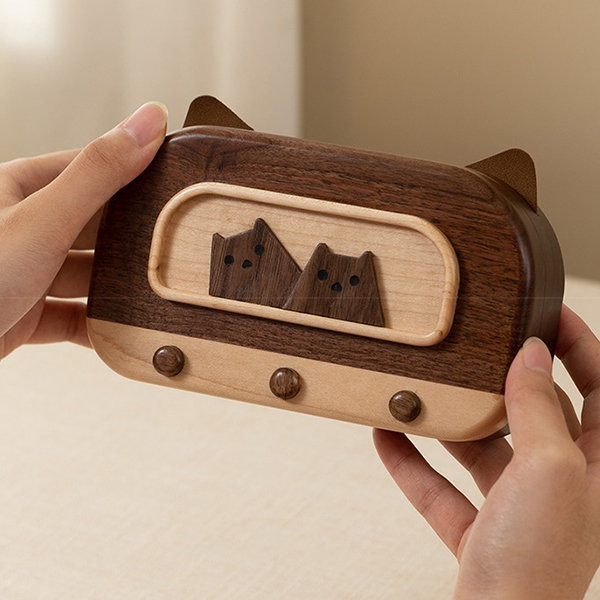In this image, a pair of hands delicately cradles a small, intricately designed wooden object, resembling a handheld video game console. The object is primarily made of dark brown wood, with a lighter wooden segment constituting about one-sixth of the bottom. It features two small wooden ears at the top corners, matching the same wooden aesthetic. In the center of the dark portion, two animal figures—possibly cats or bears—are visible, each with distinctive black eyes and noses, appearing through what looks like a window on the device. Below these figures, three wooden buttons are neatly arranged. The background of the image is a simple, uncluttered beige.